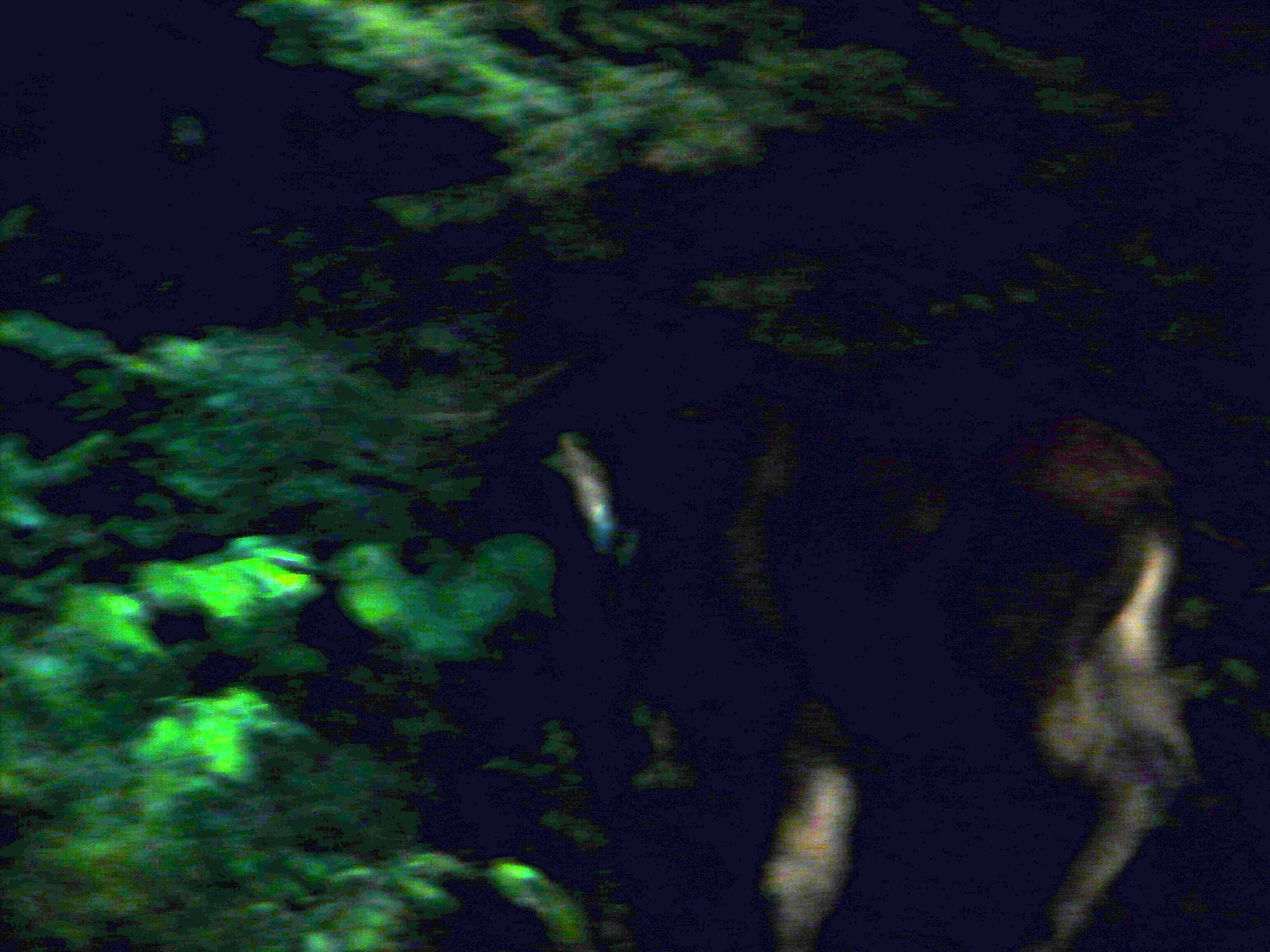The image appears to be a weather map, reminiscent of those shown on The Weather Channel, illustrating meteorological data over a geographic region. The map prominently features large, irregularly shaped green areas, likely representing precipitation patterns, superimposed on a blue background, which might symbolize the ocean or a significant body of water. The left side of the image is dominated by a bright green mass, indicating heavy rainfall or dense cloud cover. In contrast, the right side has a smaller, beige-colored area, possibly denoting a landmass or a dry region. The image effectively depicts the contrast between the wet, stormy left section and the drier, possibly land-based right section.